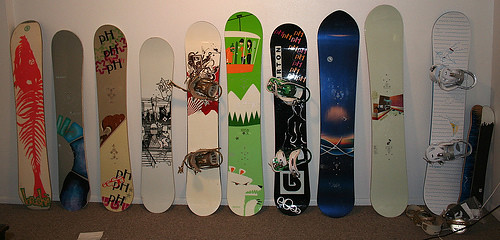The image captures an array of ten snowboards of varying heights and designs, all leaning neatly against a white wall. They rest on a short, flat, brown carpet, creating a contrasting backdrop. Among them, three snowboards are equipped with metal foot attachments, setting them apart. The designs on the boards range widely: one features a cream-colored background with a red fish skeleton design, another is blue and gray, and one has green illustrations depicting snowy mountains and people on a ski lift. The central board, without foot attachments, stands out with its polar bear design and snowy mountain motif. Some other notable designs include a board with an outer space theme and another with white stripes. Each snowboard showcases a distinct artistic style, making the collection visually captivating.